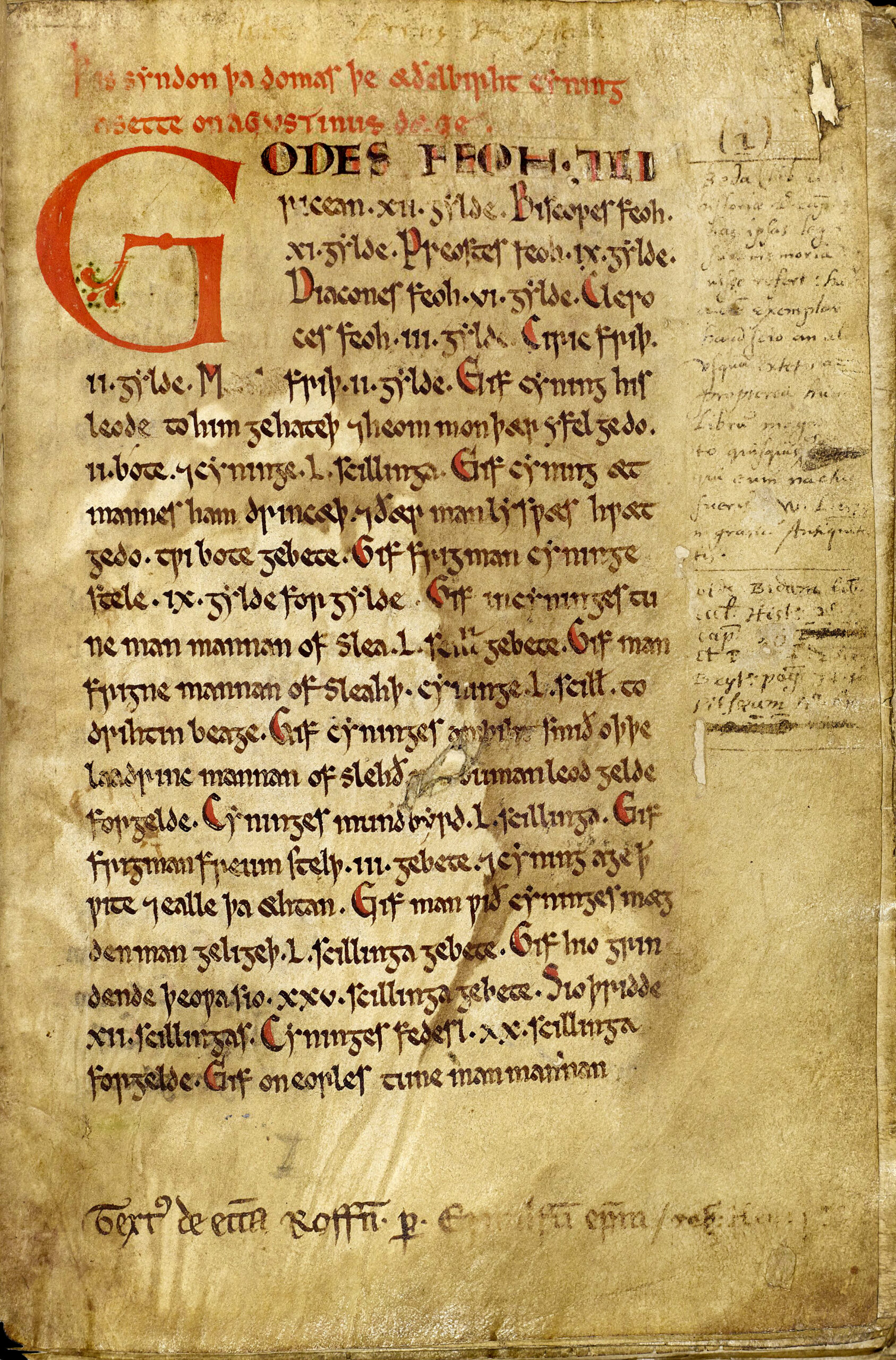The image is a vertical, rectangular depiction of an old, realistic-looking piece of parchment, possibly a scan or photograph. The parchment is beige with darker gray and tan patches, indicating age and wear, with edges darkening and sporting occasional holes and tears, including a significant one on the right-hand side that resembles a burn mark. Across the top, there is faint red text, along with a large, fancy red letter "G" on the top left. Below this, a main paragraph of black text runs down the page, interspersed with red-highlighted capital letters, while a smaller column of handwritten notes and scribbles appears to the right. This text appears similar to English but is in an unfamiliar language. The document concludes with a worn footer, the text fading to the point of illegibility as it reaches the bottom.